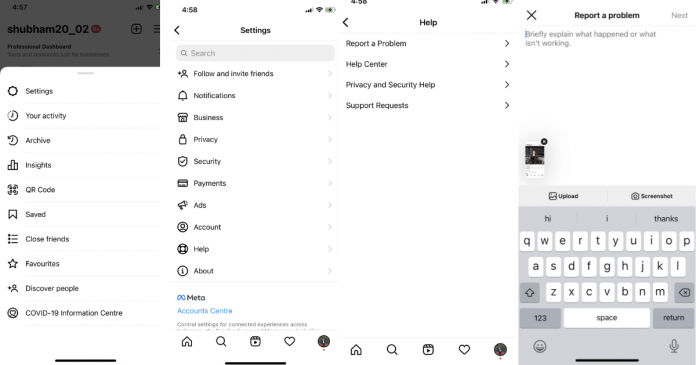A series of four smartphone screenshots outlines the step-by-step process to report an issue on an application. 

**Screenshot 1**: The first image displays the user interface of the app, showing the profile page of user "Shubham20_02" on Instagram. Multiple options are listed, including "Settings," "Archive," "QR Code," "Close Friends," "Favorites," "Discover People," and "COVID-19 Information Center." The highlighted option is "Settings."

**Screenshot 2**: In this image, the user has navigated to the "Settings" menu. This menu includes various options such as "Follow and Invite Friends," "Notifications," "Business," "Privacy," "Security," "Payments," "Ads," "Account," "Help," and "About." The selected option here is "Help."

**Screenshot 3**: The third screenshot shows the "Help" submenu with four choices visible: "Report a Problem," "Help Center," "Privacy and Security Help," and "Support Requests." The user has selected "Report a Problem."

**Screenshot 4**: The final screenshot captures the screen after selecting "Report a Problem," where a keyboard has appeared, allowing the user to type the details of the issue they wish to report.